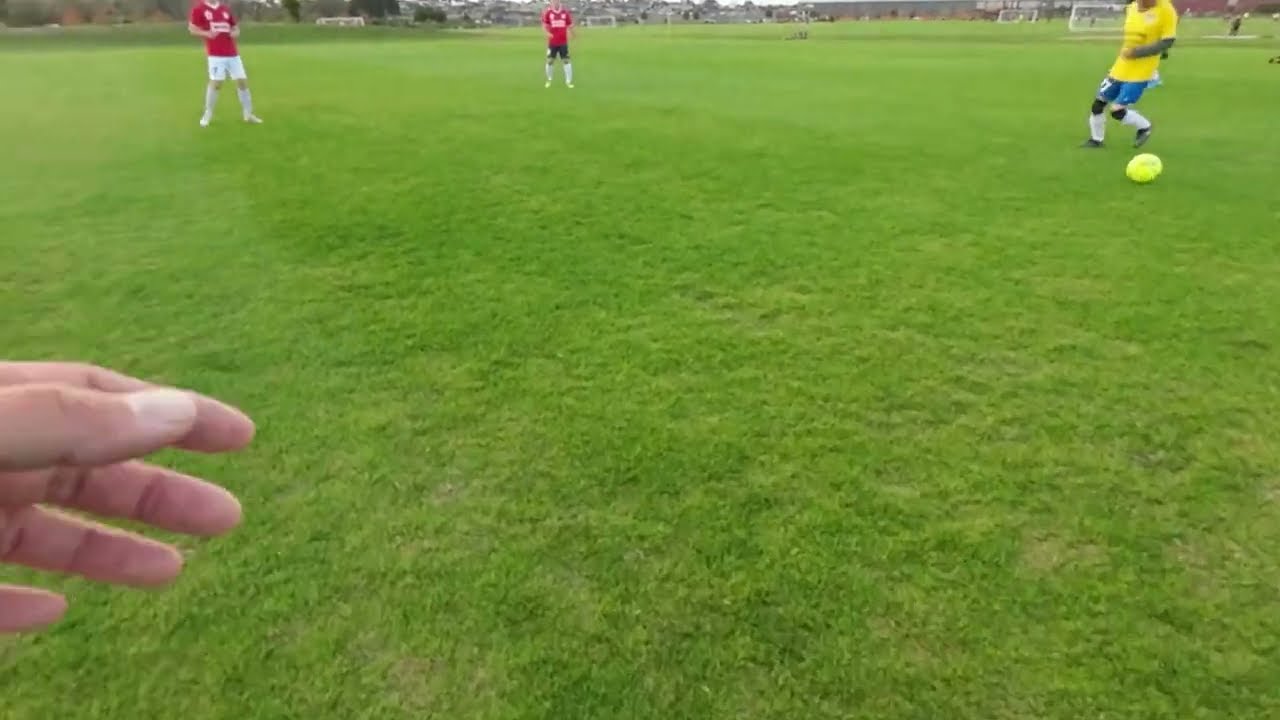In this first-person perspective photograph taken on a grassy soccer pitch, the photographer’s left hand is visible at the bottom left of the image. Dominating the scene are three players on the field. On the right, a player dressed in the iconic Brazil colors of a yellow jersey and blue shorts is handling a neon green ball. At the center left, another player stands with his hands behind his back, wearing a red jersey and white shorts. To the far left of the image, a third player also dons a red jersey. The background features soccer nets, hinting at a practice session on an unlined section of the field. The image, taken outdoors during the day, captures vibrant colors with various shades of green grass, along with red, yellow, blue, white, tan, and black elements.